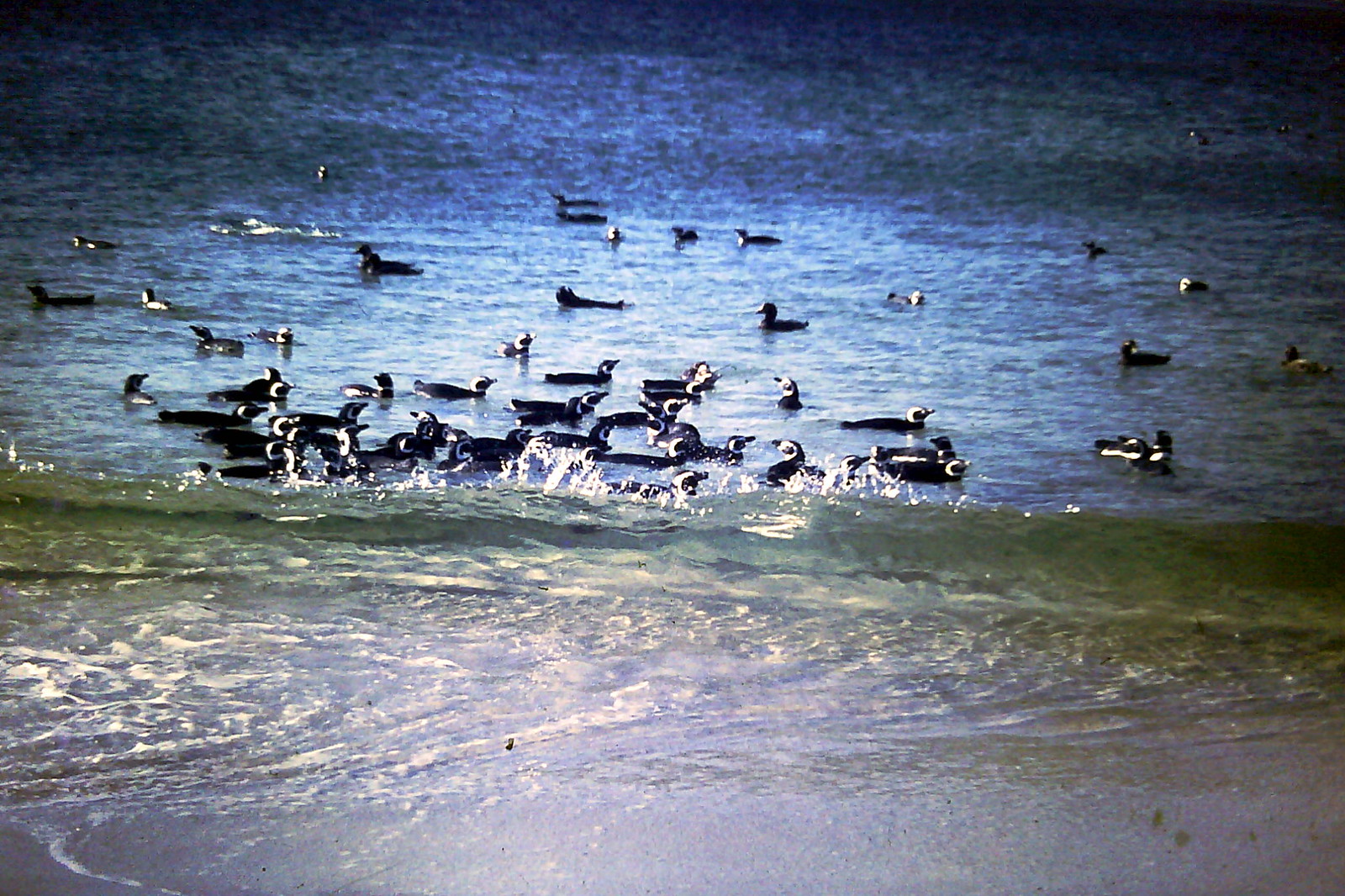The photograph is a rectangular outdoor scene taken during the daytime, approximately four inches tall and six inches wide, looking out over an expansive ocean area. The lower half of the image shows the ocean meeting a sandy shore, where almost clear green waves transition to an ambery blue-white as they wash over the sand. The crests of the waves are adorned with white foam tips. Beyond the greenish water near the shore, the ocean transitions from light blue in the center to a darker navy blue further out. Throughout the water, numerous aquatic birds float on the surface. These birds appear to be black ducks with distinctive white head markings that form a C-shape around their heads and chins, with the black located towards their beaks. The birds' backs are plain black. Despite the photo's slight graininess, it is clear that the birds are intermingling closely and navigating the choppy water, which shows white caps especially towards the foreground. The water's colors vary from a brownish-green near the front to a more bluish-gray towards the back, reflecting either the sun or some other light source. The image captures a dynamic and serene seascape populated with duck-like birds, contributing to a detailed and vibrant coastal scene.